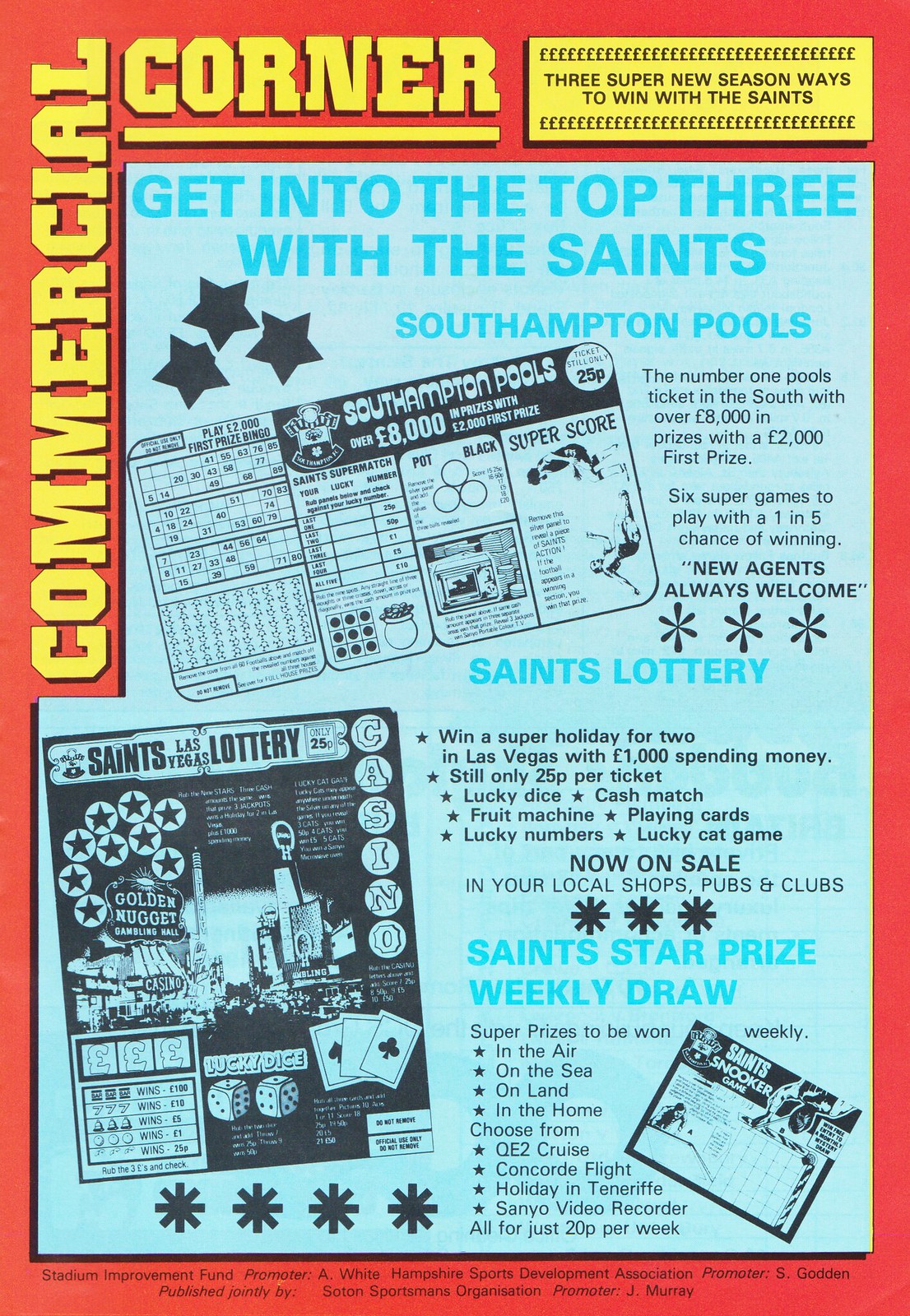The image is an advertisement, likely from a magazine, featuring a red background and the words "Commercial Corner" in yellow on the upper left. The ad prominently highlights "Three Super New Season Ways to Win with the Saints." At the center, against a light pale bluish-white background, the text reads "Get into the Top Three with the Saints," followed by "Southampton Pools, Saints Lottery, Saints Star Prize, Weekly Draw." It includes visuals related to lottery tickets and pools, and additional small print at the bottom. The border of the central section is red, and there's a note mentioning "New Agents Always Welcome" with asterisks scattered throughout the page.